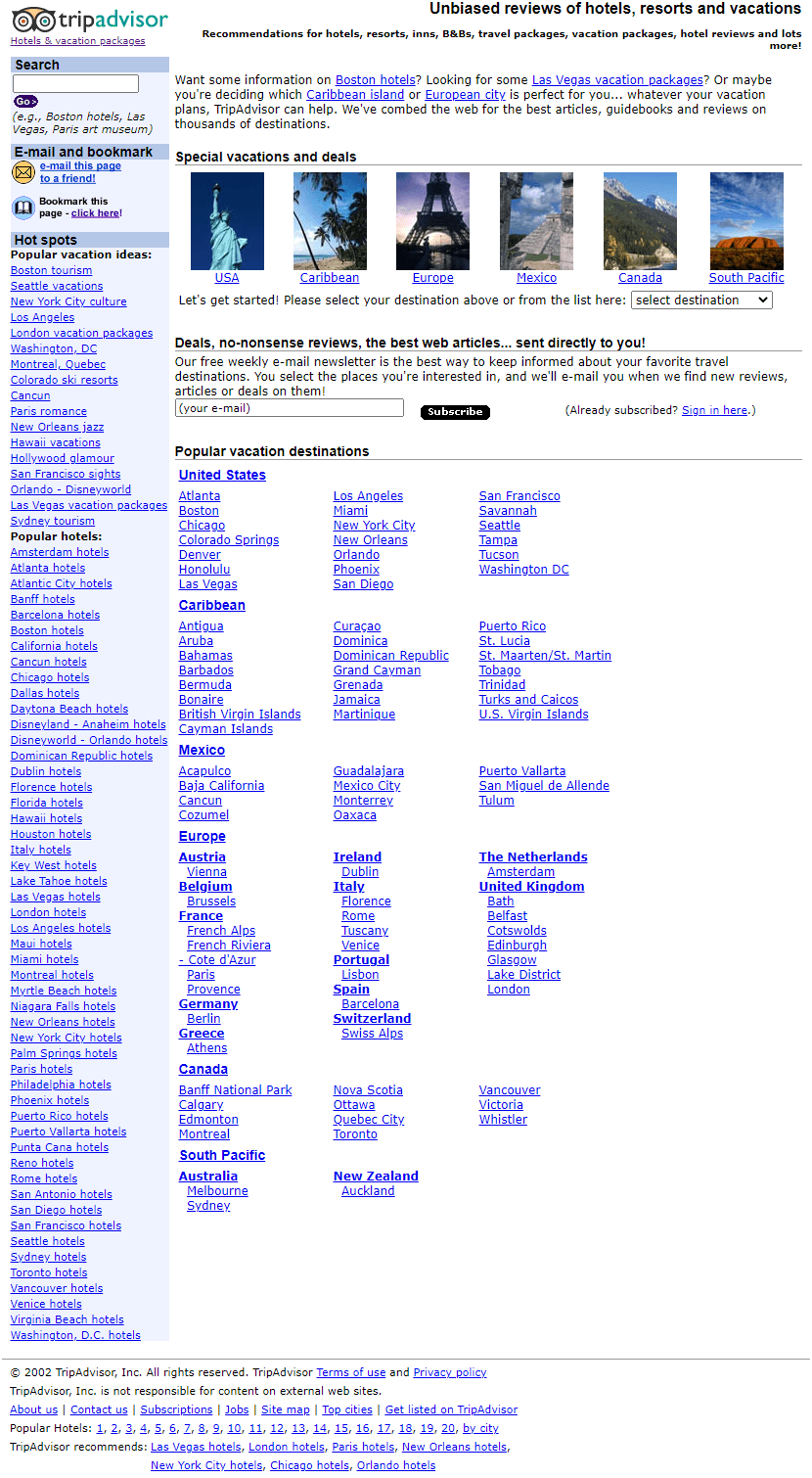On a clean white background, the prominent TripAdvisor logo stands out. The word "Trip" is displayed in black, while "Advisor" appears in a teal color. The logo features an owl with two eyes resembling binoculars, symbolizing detailed and watchful reviews. Below the logo, the tagline reads, "Unbiased reviews of hotels, resorts, and vacations."

A blue rectangle with the word "Search" written in black provides a prompt for users. Adjacent to it, a search bar is readily available for entries. Additional options such as email, bookmarks, and information are highlighted in blue.

Highlighted sections labeled "Hot Spots," "Popular Vacations," and "Special Deals" provide further details. Popular destinations listed include the USA, Caribbean, Europe (or more specifically, possibly France), along with others that start with the letters "M" and "C," and the South Pacific.

The layout, designed with user-friendliness in mind, helps visitors quickly find relevant travel information and deals.